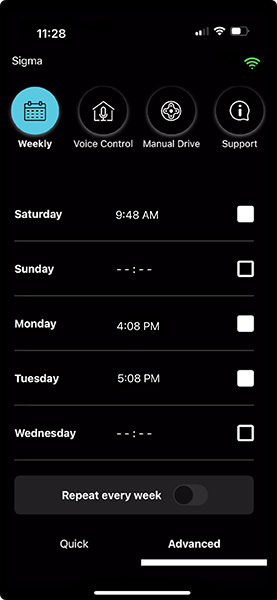This is a clear screenshot taken from an Android device. The background is pitch black. At the very top-left corner, in white letters, 11:28 is displayed, indicating the time. On the top right, there are various status icons: 2 out of 4 signal bars, a Wi-Fi symbol, and a half-full battery icon in white. Just below these icons, in the upper-left corner, the word “Sigma” is visible in white letters.

On the far top-right, there is another green Wi-Fi symbol. Below these elements, there are four clickable icons. The first icon on the left is an aqua blue circle with a black calendar symbol inside it, labeled “Weekly” in white letters underneath. 

The second icon from the left is a black circle with a white outline, containing a house symbol with a microphone at the center. It is labeled “Voice Control” underneath. 

The third icon is a black circle with a white outline, and inside it is a white game controller icon. It is labeled “Manual Drive” underneath.

The fourth, and rightmost icon, is a black circle with a white outline featuring a speech bubble with a lowercase letter “i” inside. It is labeled “Support” underneath.

Below these icons, several rows are separated by gray bars. The first row has “Saturday” at the left, "9:48 AM" in the middle, and a filled white square on the far right. 

The next row has “Sunday” on the left with two dash-dot symbols, and on the right of it, an unchecked black-filled box.

The "Monday" row is in white letters with “4:08 PM” written in the middle and a filled white square to the right. 

The "Tuesday" row has “5:08 PM” at the center with another filled white square to the right. 

The "Wednesday" row has dash-dot symbols at the center with an unchecked black-filled box to the right. 

Below these rows, a long gray bar displays the text “Repeat Every Week” in white letters, and beside it, a black circle toggle is positioned toward "Repeat Every Week."

Lastly, beneath this toggle, the words “Quick” and “Advanced” are written in white letters on the left and right, respectively. At the bottom-center of the screen, there is a long white bar.